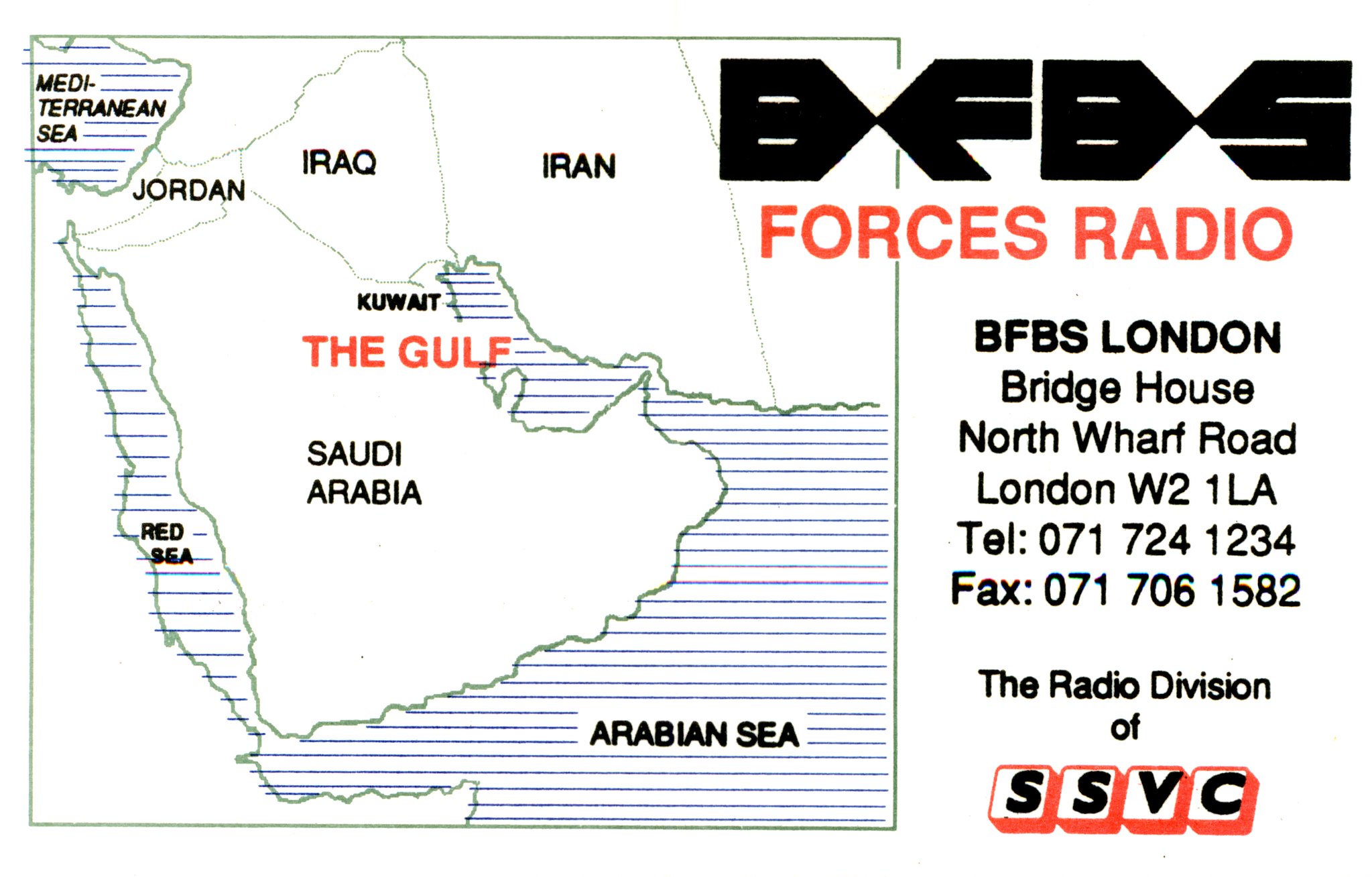The image displays a square map on the left side, depicting the Mediterranean Sea, the Red Sea, and the Arabian Sea, along with the countries situated between them, including Kuwait, Saudi Arabia, Iraq, Jordan, and Iran. The map also labels the area as "the Gulf." On the right side, the letters "BFBS Forces Radio" and "BFBS London" are prominently displayed. Beneath this, the address "Bridge House, North Wharf Road, London, W21LA" is listed, along with a telephone number (071-724-1234) and a fax number (071-706-1582). This information is presented simply, in black text on a mostly white background, indicating that it belongs to the radio division of SSVC.